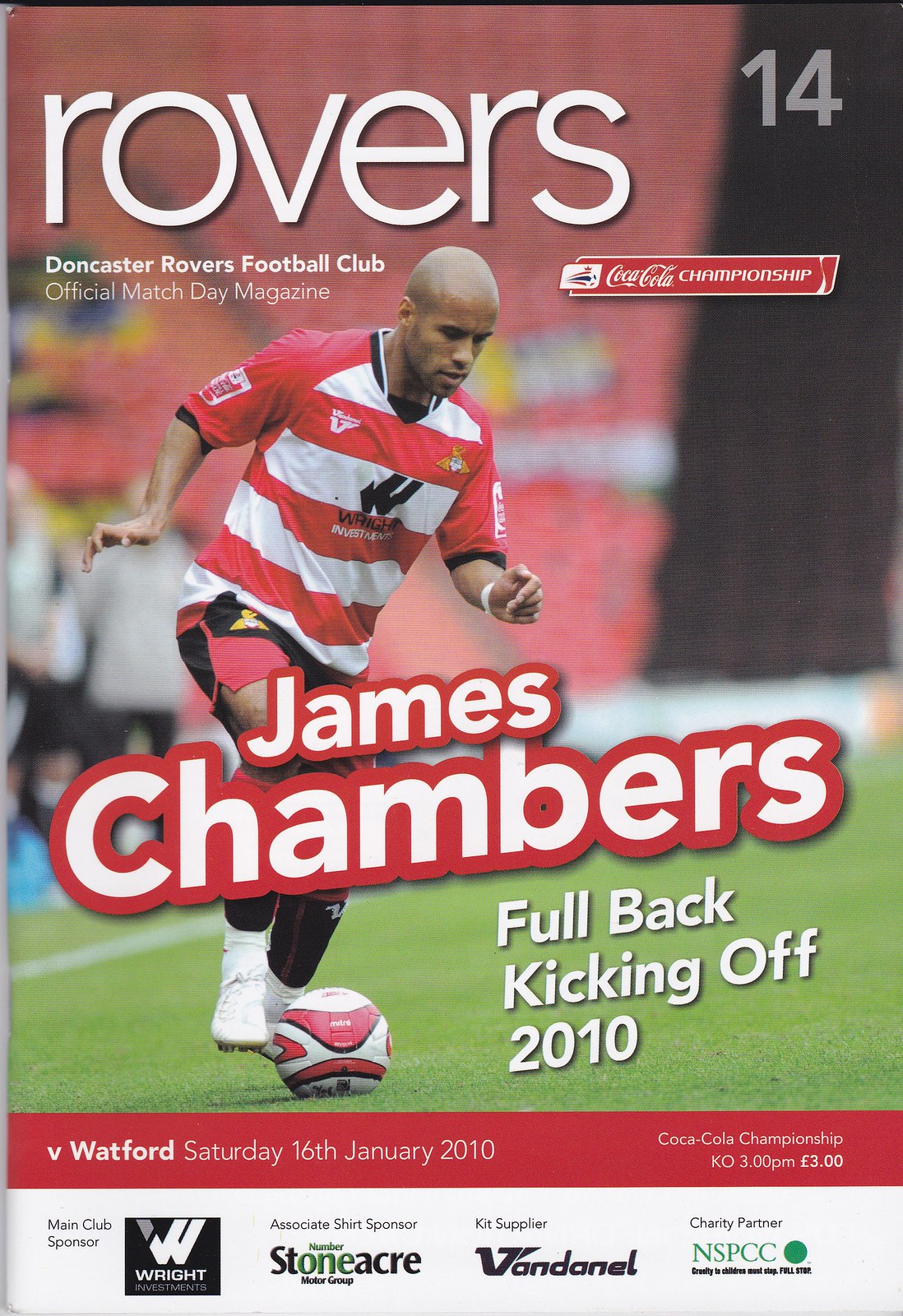The image is a vertically oriented magazine cover featuring a bald soccer player, James Chambers, who is a fullback for the Doncaster Rovers Football Club, kicking off the 2010 season. Chambers, a dark-skinned man, is depicted in action, wearing a red and white horizontal striped jersey, red and black shorts, and white cleats as he kicks a red and white soccer ball. At the top of the cover, the magazine title "Rovers" is displayed in white lettering, with "Doncaster Rovers Football Club" written underneath. The central text, in a mix of white and red lettering, prominently features "James Chambers" with the subheading "Fullback kicking off 2010." The upper right corner shows the number 14, and nearby, there is an advertisement for the Coca-Cola Championship. At the bottom, a series of sponsors are listed, including Wright Investments, Stoneacre, Vandernal, and the charity NSPCC. The cover also mentions that this edition is the official match day magazine for the game against Watford on Saturday, January 16, 2010, with a kickoff at 3 p.m., and is priced at three pounds.